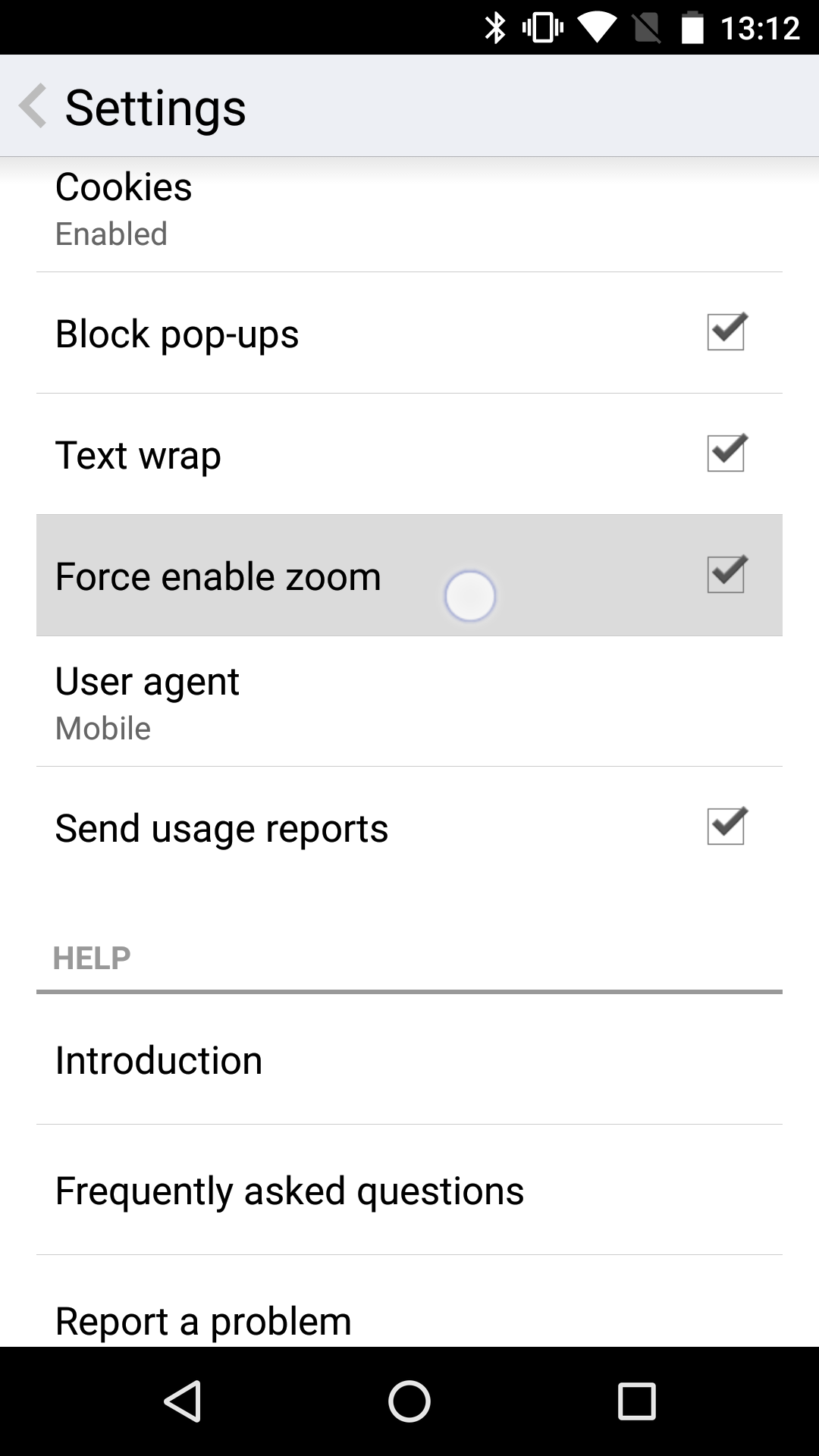This screenshot captures a detailed view of a settings window, likely from a mobile application or device, showcasing various options for configuring the system. In the upper-left corner, the title "Settings" is prominently displayed, accompanied by a left arrow pointing back to the previous menu.

Below the title, the first category listed is "Cookies," with the status indicated as "Enabled." The next option, "Block pop-ups," features a checkbox on its right side, which is currently checked off.

Following this, the "Text wrap" option also has a checked-off checkbox beside it. Further down, the "Force enable zoom" option is highlighted; its checkbox is checked off and is dark gray, signifying that a white circular cursor is currently hovering over it.

Continuing the list, the "User agent" setting displays "Mobile" within the same line as its label. Beneath this, the "Send usage reports" option appears, also accompanied by a checked-off checkbox.

The next section, denoted by the header "Help," includes three sub-options: "Introduction," "Frequently Asked Questions," and "Report a problem."

At the very bottom of the window is a navigation bar with three buttons: a back button on the left, a home button in the form of a circle positioned centrally, and a minimize button represented by a square on the right.

Additionally, the top status bar displays several icons: a Bluetooth icon on the far left, followed by a vibrate mode icon, a signal strength icon fully filled, a no SD card icon, a nearly full battery icon, and the time, which reads 13:12.